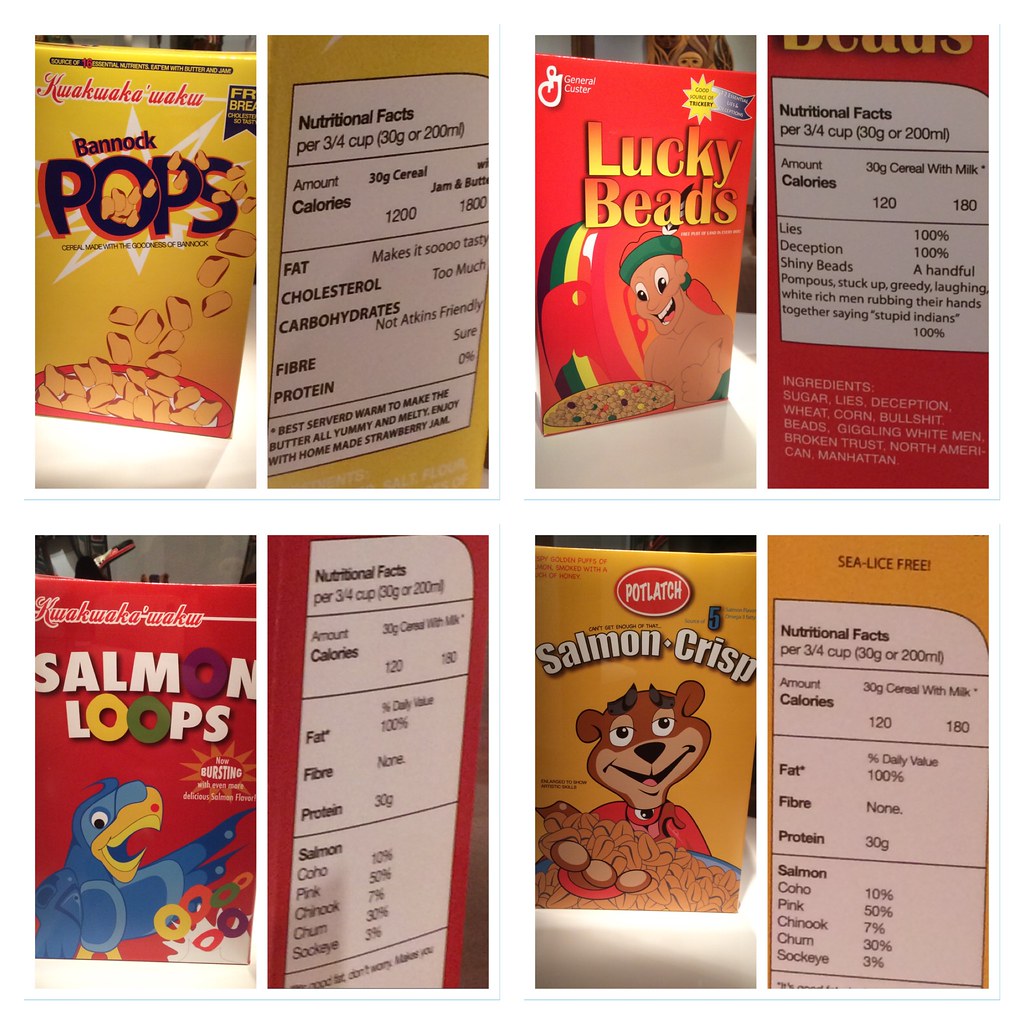The image consists of four distinct panels, each showcasing a different type of cereal box along with its nutritional facts. 

1. **Bannock Pops**:
   - **Color Scheme**: Predominantly yellow with black accents.
   - **Details**: The cereal box prominently features the name "Bannock Pops" in a bold font. Nutritional facts are displayed on the side panel, written in black.

2. **Lucky Beads**:
   - **Color Scheme**: Primarily red with a colorful rainbow.
   - **Details**: This cereal box features an animated character with an orange ponytail and a green headband. The name "Lucky Beads" is highlighted along with the colorful rainbow. The side panel shows the nutritional facts.

3. **Salmon Loops**:
   - **Color Scheme**: Yellow and green, with an orange "O" in the title.
   - **Details**: The title "Salmon Loops" incorporates an orange-colored "O" and the rest of the lettering in yellow and green. The front of the box depicts a blue bird with cereal loops resembling Fruit Loops flying out of it. The nutritional facts are indicated on the accompanying panel.

4. **Salmon Crisp**:
   - **Color Scheme**: Mainly yellow.
   - **Details**: This cereal box features a brown bear as its mascot. The name "Salmon Crisp" is prominently displayed. The nutritional facts are provided on the side panel.

Each illustration provides a clear representation of the cereal's branding, the character or mascot associated with it, and a dedicated section for the nutritional information.